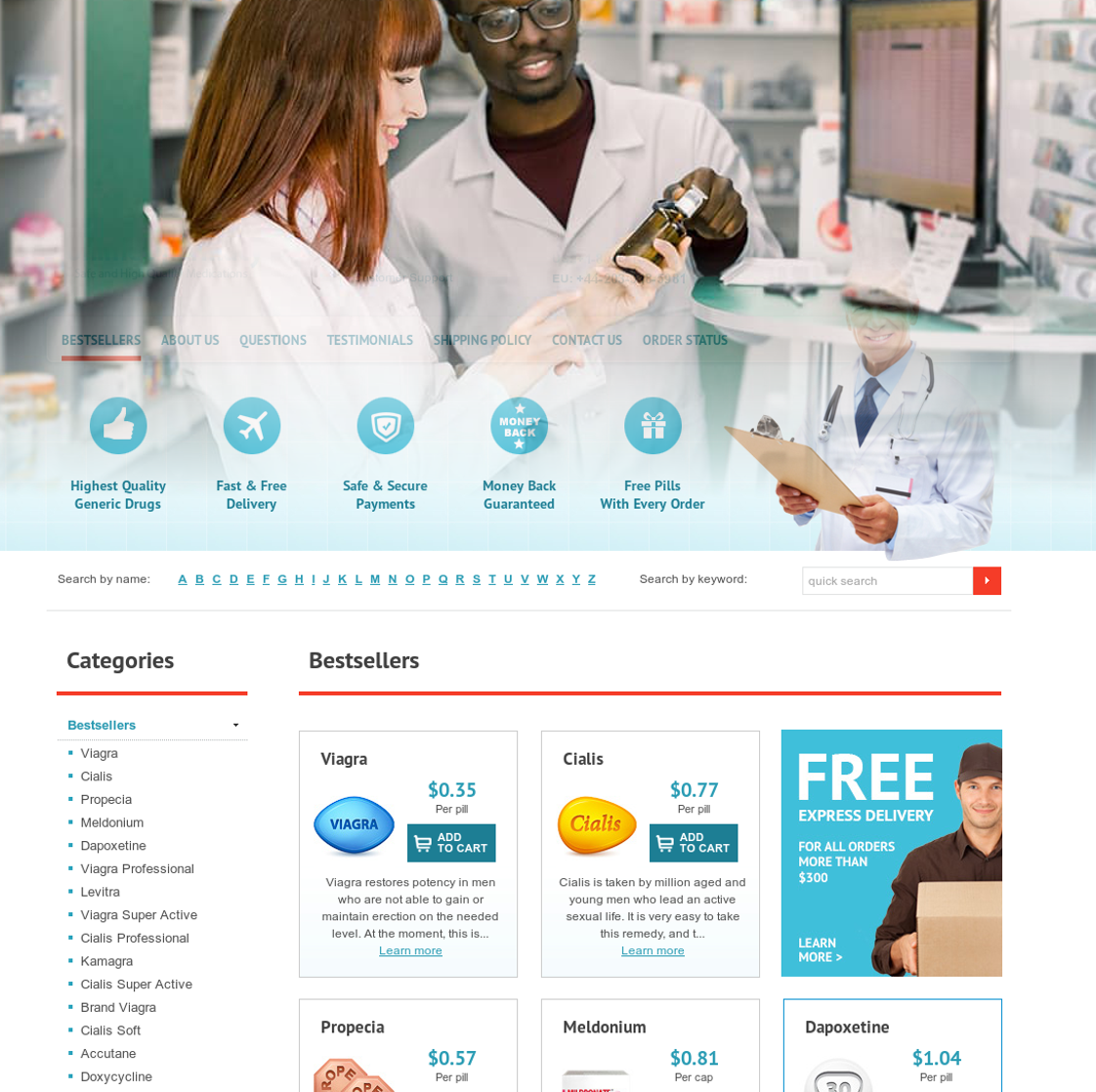The website image showcases a professional and user-friendly interface focused on a medical and pharmaceutical theme. At the top of the page, a large background image features a man and a woman, presumably pharmacists, working inside a pharmacy. Overlaying this background are horizontal navigation options in all capital letters: "BEST SELLERS" (underlined with red), "ABOUT US," "QUESTIONS," "TESTIMONIALS," "SHIPPING POLICY," "CONTACT US," and "ORDER STATUS."

Below the navigation bar, there are graphical icons with text that highlight key features of the website: "Highest Quality," "Generic Drugs," "Fast and Free Delivery," "Safe and Secure Payments," "Money Back Guarantee," and "Free Pills with Every Order."

The background then shifts to white, introducing sections for "Search by Name" with an alphabetically arranged interface and "Search by Keyword" accompanied by a search bar labeled "Click Search."

On the left side, a section titled "Categories" (underlined with red) lists various drug categories. Adjacent to this, another section titled "Best Sellers" (also underlined in red) displays several product squares, each featuring the drug's name and a brief description.

Additionally, there is a prominent banner that advertises "Free Express Delivery," emphasizing the efficiency and customer-friendly policies of the service.